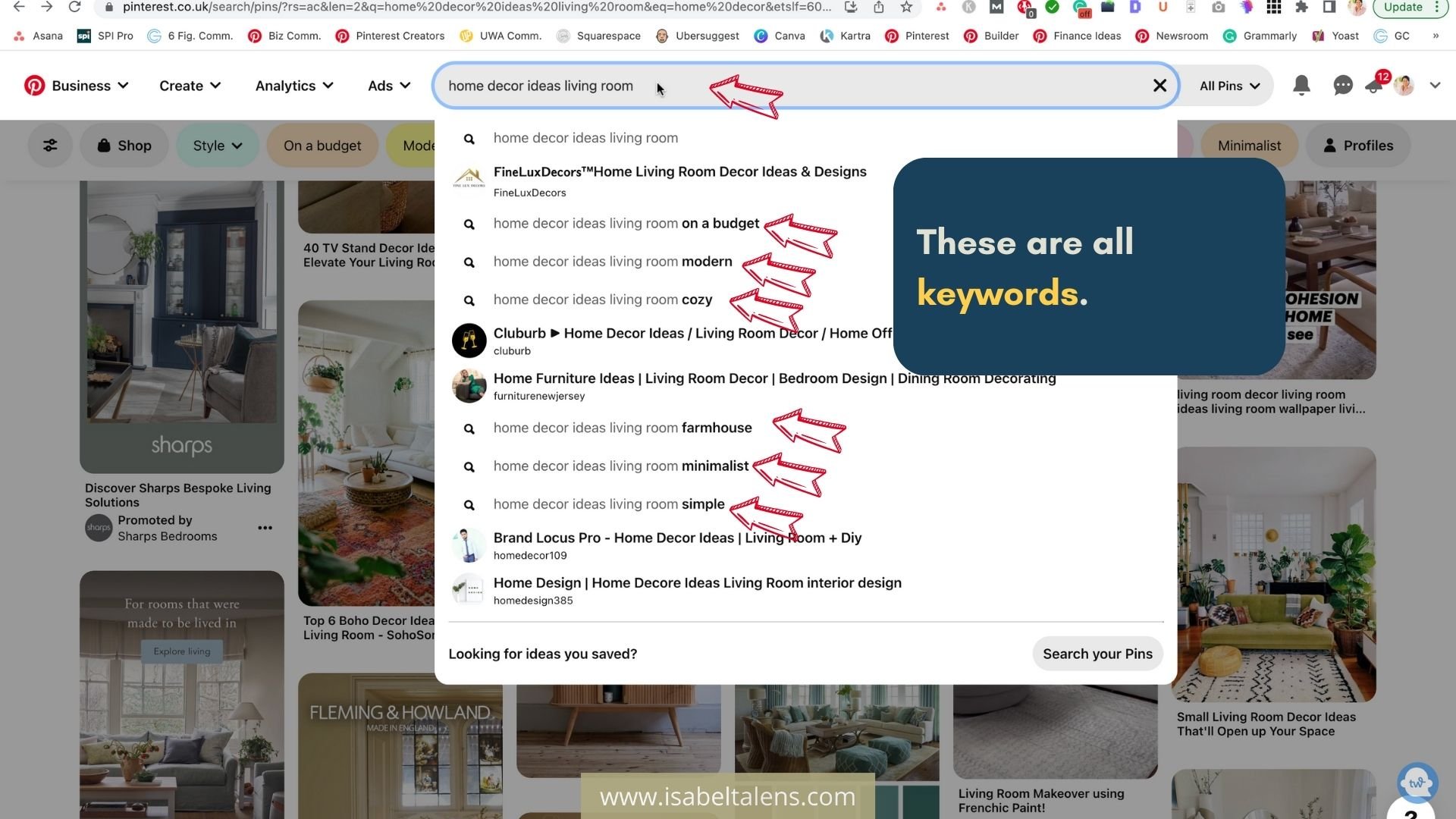The image is a detailed screenshot of a search result for the term "Home Decor Ideas Living Room". The search term is typed into the search box, triggering a drop-down menu filled with search suggestions. An overlay image with text has been added, indicating these suggestions as keywords. The keywords identified include "On a Budget," "Modern," "Cozy," "Farmhouse," "Minimalist," and "Simple." These keywords stand out as they are highlighted in a darker or bolder text compared to the rest of the text in the suggestions. Illustrative arrows, seemingly drawn or inserted using a paint program, point towards these keywords for emphasis. For example, the first search suggestion reads, "Home Decor Ideas Living Room On a Budget," with "On a Budget" highlighted boldly, marking it as the keyword. Similarly, another suggestion highlights "Modern" in "Home Decor Ideas Living Room Modern," underscored by its bolder font, signifying its importance as the keyword.